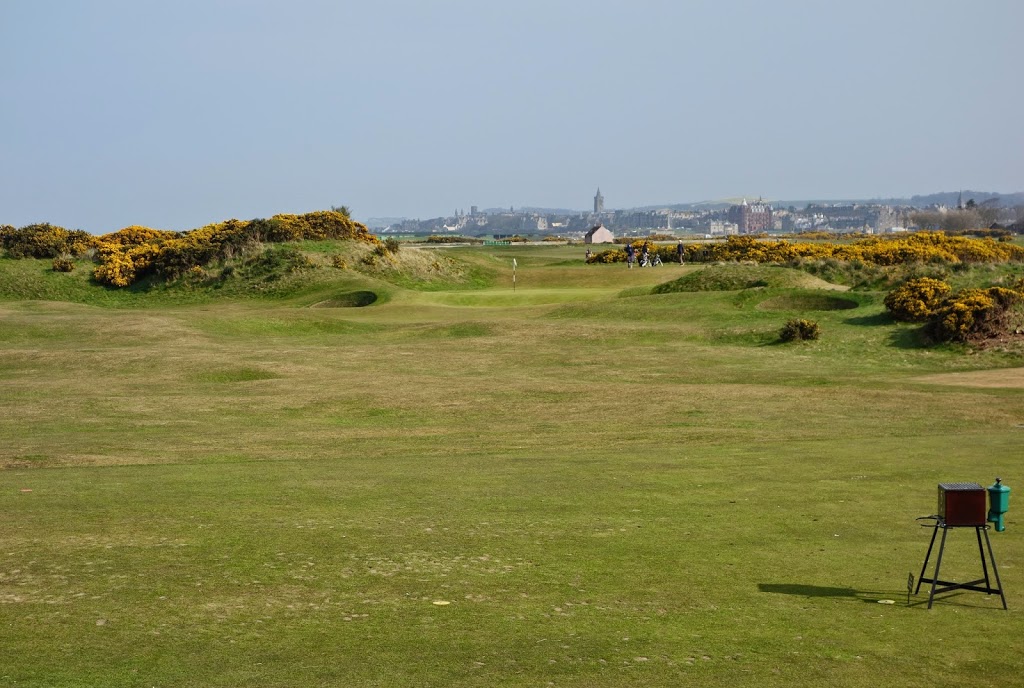This image captures a sprawling, lush green landscape that resembles a golf course, complete with undulating terrain, holes in the lawn, and several patches of brown and yellow grass. The top of the scene features a clear blue sky. The midsection of the image, towards the right, is dotted with a variety of tall, stone buildings reminiscent of a European city, possibly London, characterized by their towers and varying hues of red, white, tan, and gray. In the distant background, there's a black and white striped golf flag marking a hole, surrounded by people either playing or watching golf.

In the foreground, particularly in the bottom right corner, stands a vintage-looking barbecue pit or table – a brown wooden box perched on four steel legs. This box has a green lantern hanging off its side, potentially used for golf ball cleaning. The grassy area around it is interspersed with green and yellow bushes. The diverse landscape, combining both metropolitan structures and natural greenery, brings out the charm of this picturesque scene.